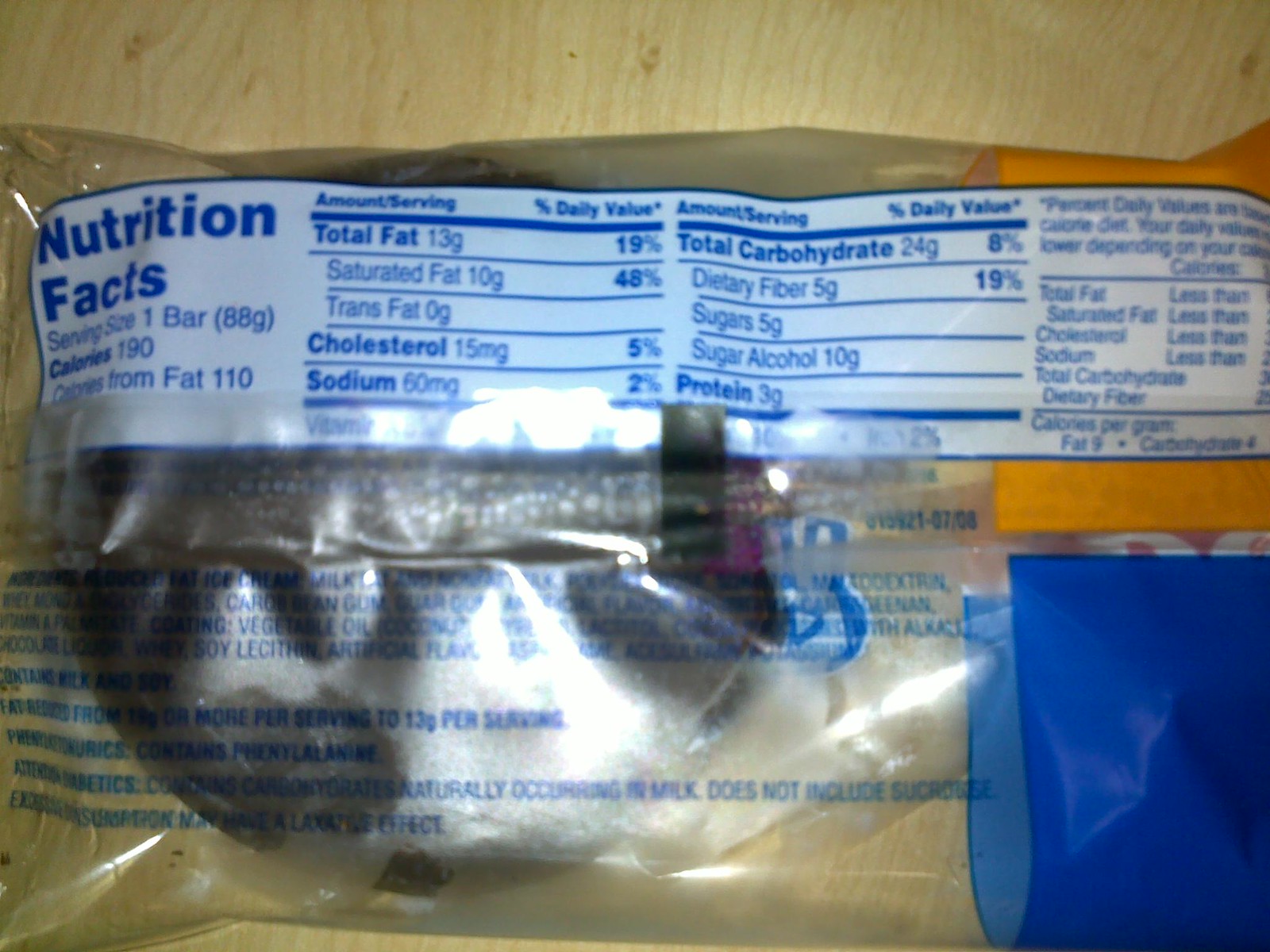The image depicts a clear plastic package of food, specifically a candy bar, lying on a brown wooden table with a visible grain pattern. The package features a nutritional facts label on the upper third, which is white with blue text. The label details a serving size of one bar, weighing 88 grams, with nutritional information stating 190 calories per bar and 110 calories from fat. Additional nutritional details include total fat at 13 grams (19% daily value), saturated fat at 48%, cholesterol at 15 milligrams (5% daily value), sodium at 60 milligrams (2%), total carbohydrates at 8%, and dietary fiber at 19%. The rest of the package is clear, revealing more blue text providing ingredient information, and through the back, the blue General Mills logo is faintly visible. Despite the label indicating it is a bar, the item inside appears round and brown, resembling a donut or cookie.